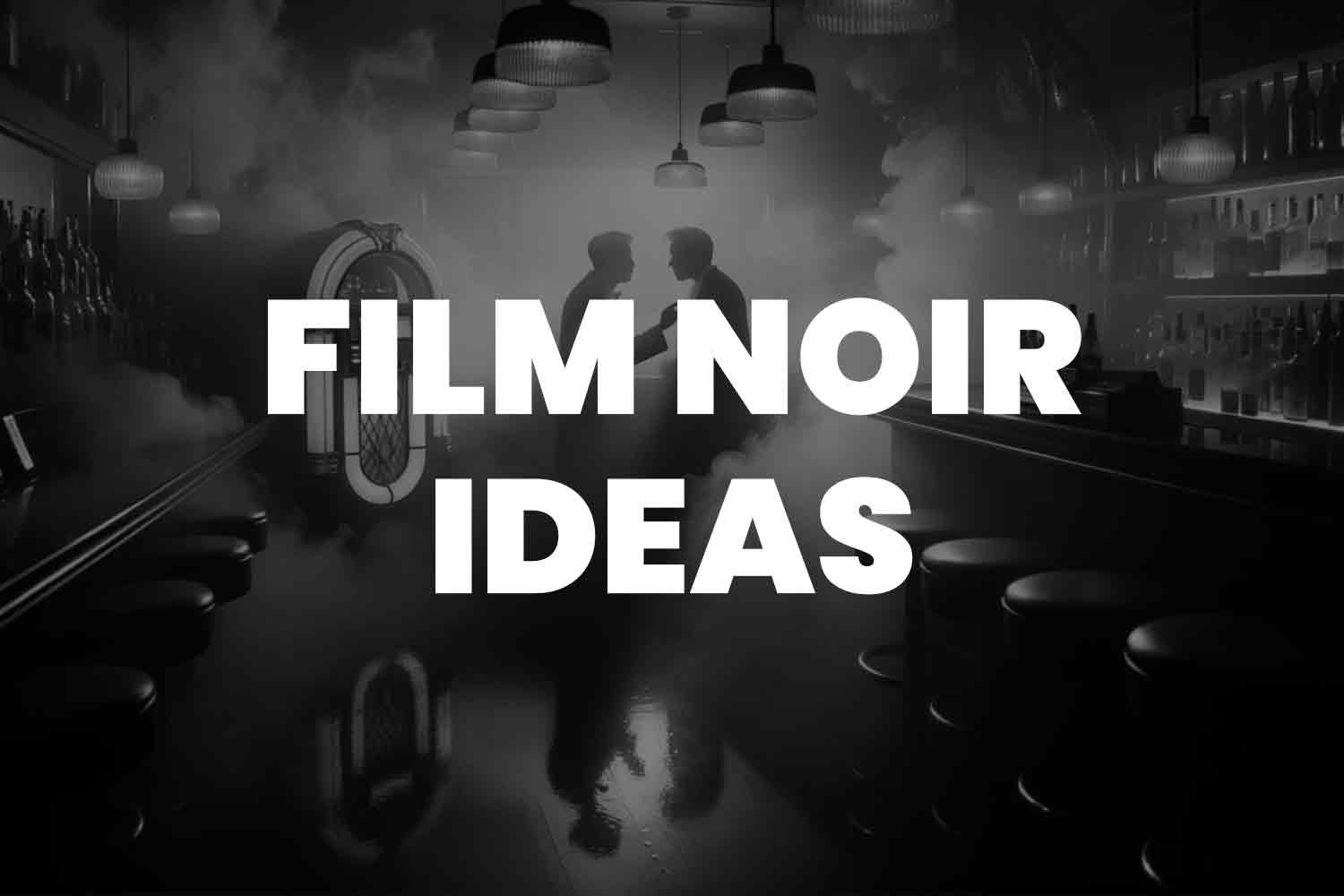In this black and white digital rendering or photo titled "Film Noir Ideas," two individuals in suits sit close together in a smoky bar setting, appearing to be in a tense confrontation. The image is dominated by large, bold white text stating "Film Noir Ideas," which prominently overlays the scene. The background reveals a dimly lit bar with vintage elements including a jukebox, whose reflection, along with those of the individuals and bar stools, is visible on the shiny, polished floor. The bar is flanked by padded stools and shelves lined with silhouetted liquor bottles. Distinctively, eight lights hang on long strings from the ceiling, adding an eerie and uneven lighting that contributes to the image's noir atmosphere. The overall scene captures a classic film noir vibe with its smoky, mysterious ambiance, enhanced by the mirrored reflections and the meticulous detail in the vintage decor.